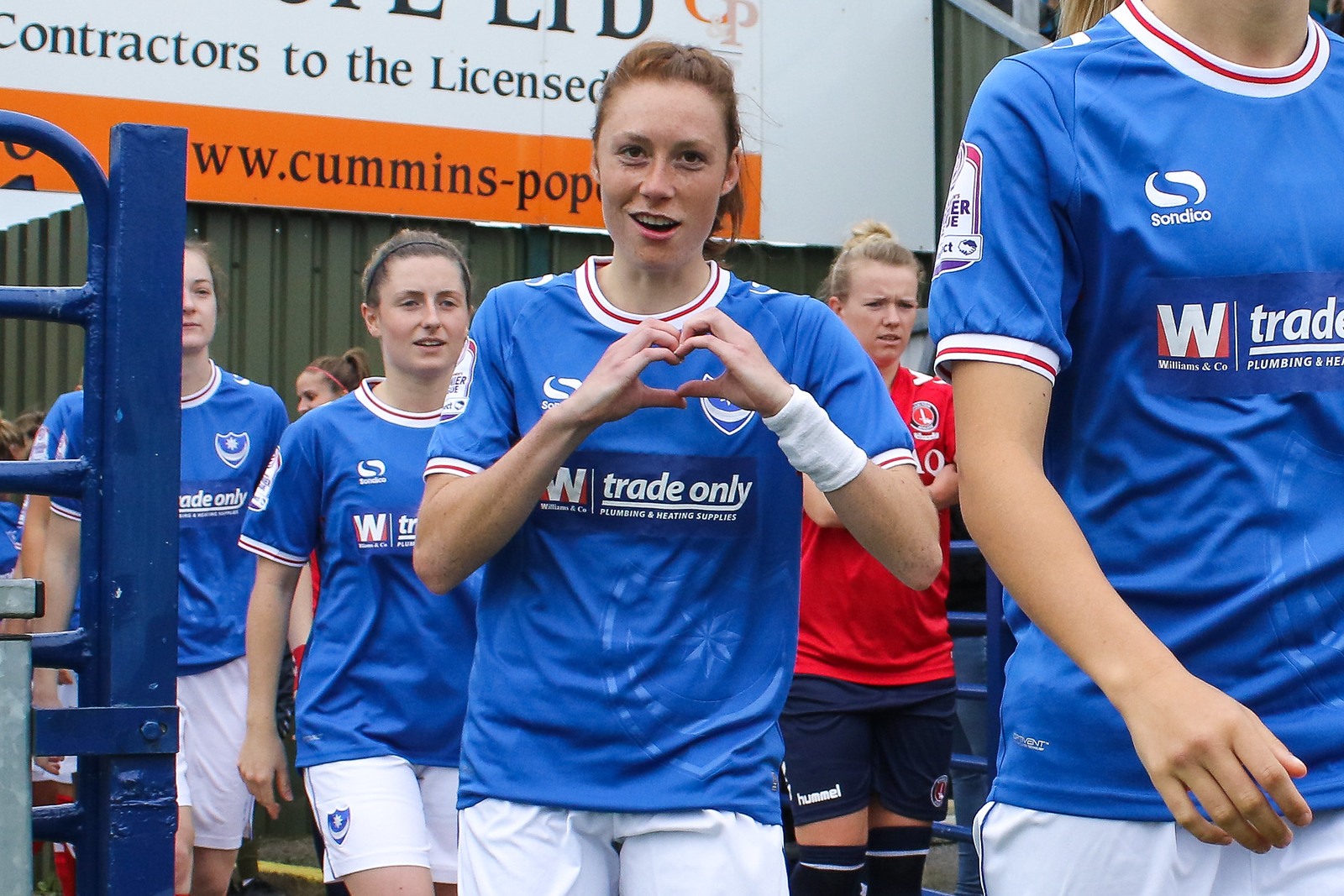The image captures a scene at an outdoor track meet featuring a group of female athletes. The focus is primarily on four runners dressed in matching blue sports tops with a prominent white "W" and the text "Trade Only Plumbing and Heating Supply." They are paired with white shorts. The figures are standing near blue gates, all with light skin and hair tied back in buns. In the background, there's a sign that reads "Contractors to be licensed, www.cummins.com." The central figure, a red-haired girl with a white wristband, is making a heart symbol with her hands and has a pleasant expression. To her right stands another athlete in a contrasting red top, black shorts, and black socks, adding diversity to the scene. Oranges, blues, and whites dominate the color palette, situating the setting clearly in a vibrant sporting event.